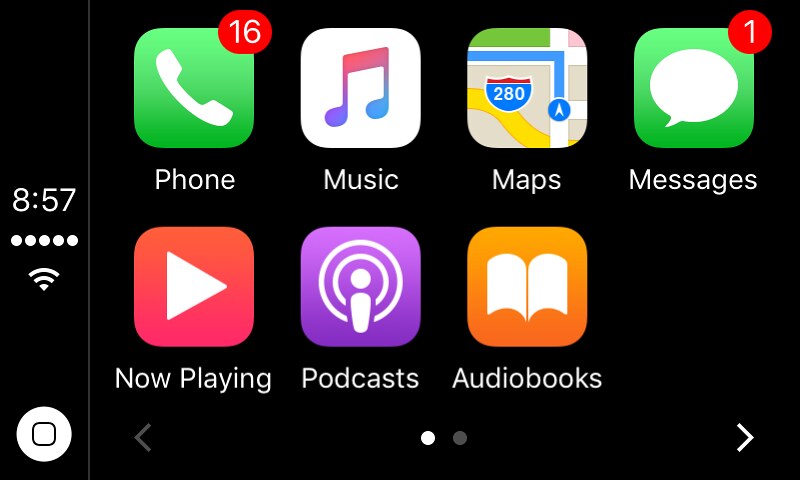The image displays a screenshot of an iPhone in landscape mode. On the left-hand side of the screen, the time is shown as 8:57, though it is not specified whether it is AM or PM. Directly below the time indicator, there are five small dots aligned horizontally. Beneath these dots is a WiFi signal icon, and at the very bottom of the left-hand column, there is a white circle containing a white square inside it.

The background of the screen is black and all text is displayed in white, creating a clear contrast. To the right of the time, seven app icons are arranged. These apps are, in order: Phone, Music, Maps, Messages, Now Playing, Podcasts, and Audiobooks.

The Phone app icon is square with rounded corners, featuring a green background and a white phone symbol. In the top right corner of this icon, a red oval badge with a white number "16" indicates there are 16 missed calls. Similarly, the Messages app icon shares the same square shape with rounded corners and a green background, displaying a white speech bubble. In the top right corner of the Messages icon, a red circular badge with a white number "1" signifies there is one unread message.